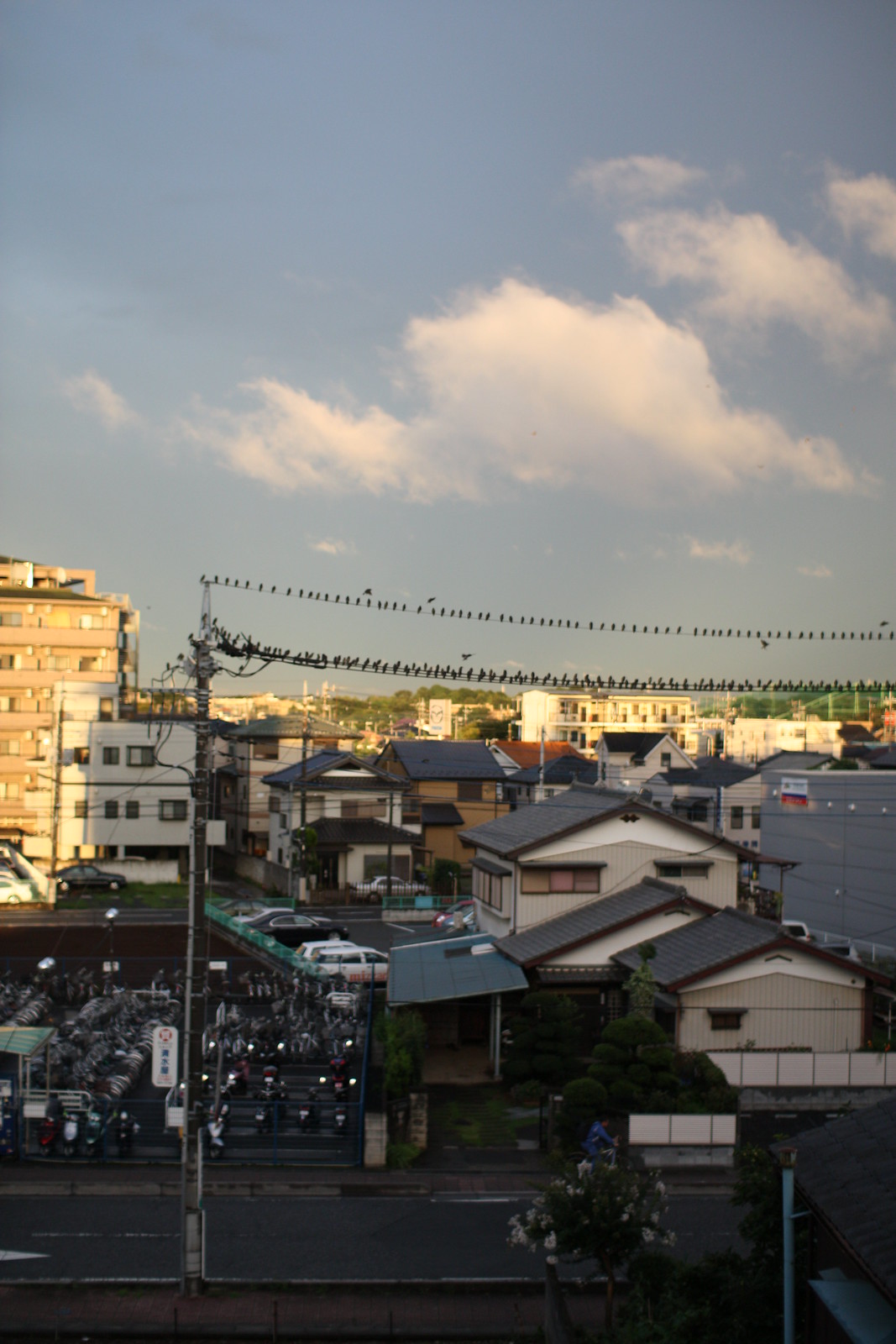The photo captures a vibrant urban scene from an elevated vantage point, possibly a balcony or hill. The sky overhead is blue with scattered white clouds, framing a cityscape below with small apartment buildings and houses. In the distance and up close, a mix of tall trees adds greenery to the environment. Prominently featured is a power line stretching across the image, both cables densely populated with small black birds perched along its entire length. Below the power lines, various streets run parallel, lined with sidewalks and small buildings. A light brown building with many windows stands out, and off to the left, there's a parking area filled primarily with motorcycles and a few cars, adjacent to a house. Further down, a person in a blue outfit rides a bike along one of the roads. The composition captures the bustling essence of city life with its mixture of natural and urban elements.